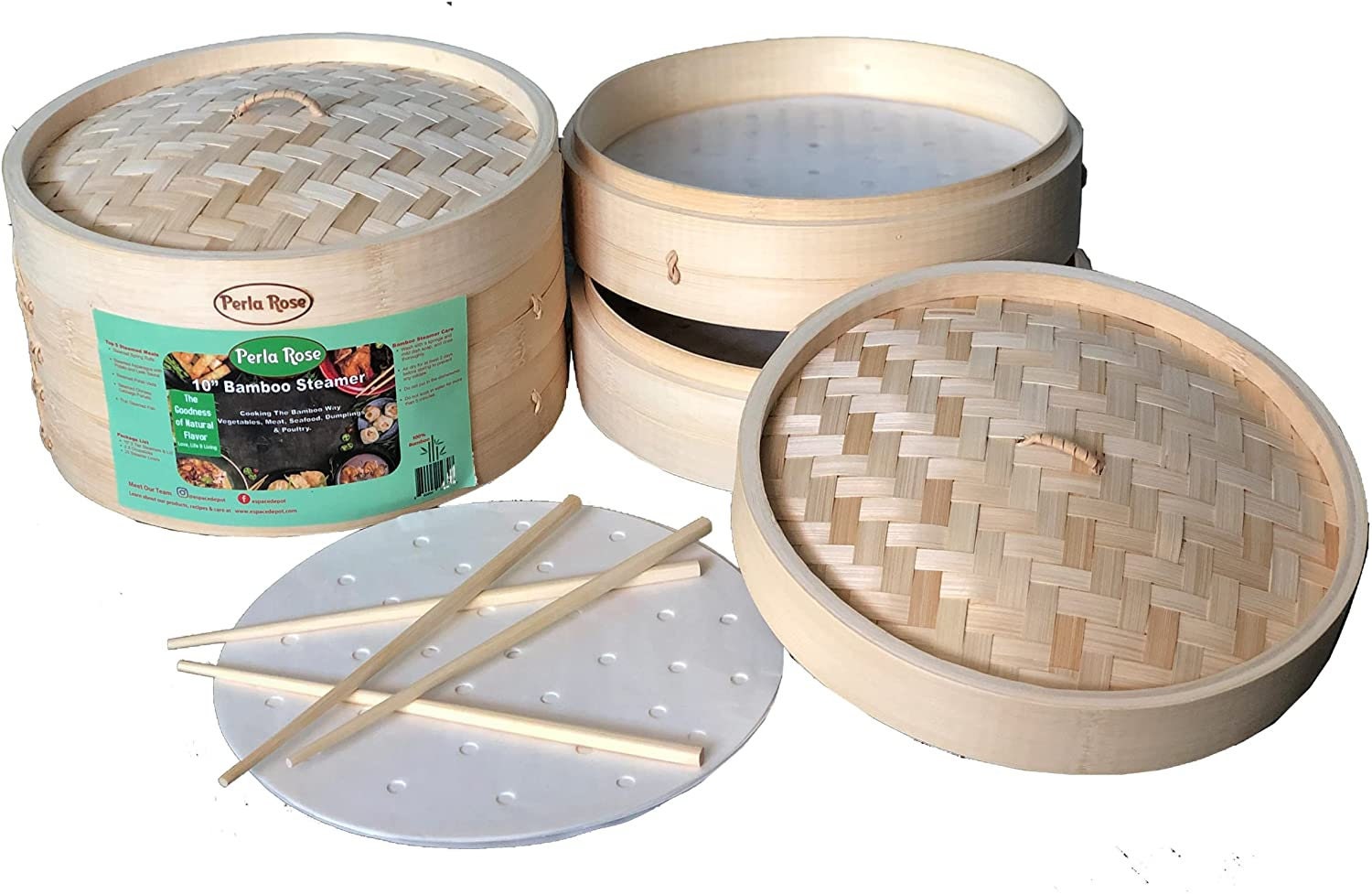The image showcases a set of two bamboo steamers, characterized by their round, woven bamboo construction. One of the steamers is opened, revealing the light-colored bamboo interior. Both lids have wicker bamboo handles for lifting. The unopened steamer features a turquoise logo from the Perlerose company, which reads "10th Bamboo Steamer" with additional information too small to be legible. Beside the two steamers, a white plastic stand displays two pairs of bamboo chopsticks. Additionally, there is a round, white filter lying between the open and closed steamers. The intricate crisscross pattern on the lids and the overall layout, including the separate compartments of the steamers, are clearly visible.